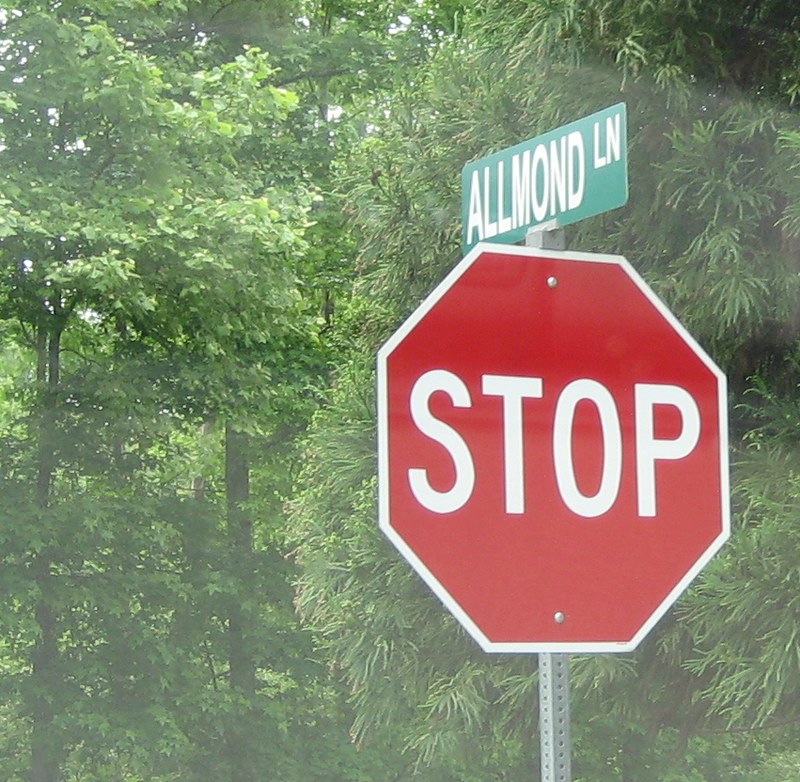The photograph captures a stop sign prominently positioned at the intersection where the viewer is situated on Almond Lane (spelled A-L-L-M-O-N-D L-N). The scene is set during late spring or early summer, evident from the lush, vibrant greenery. The background features an intriguing tree or bush resembling a spruce hedge, known for its unique needle and leaf structure. On the left side of the image, tall, narrow, old-growth trees with dense foliage stretch upwards, adding depth to the verdant landscape. The overall atmosphere is fresh and rejuvenating, embodying the essence of the season.